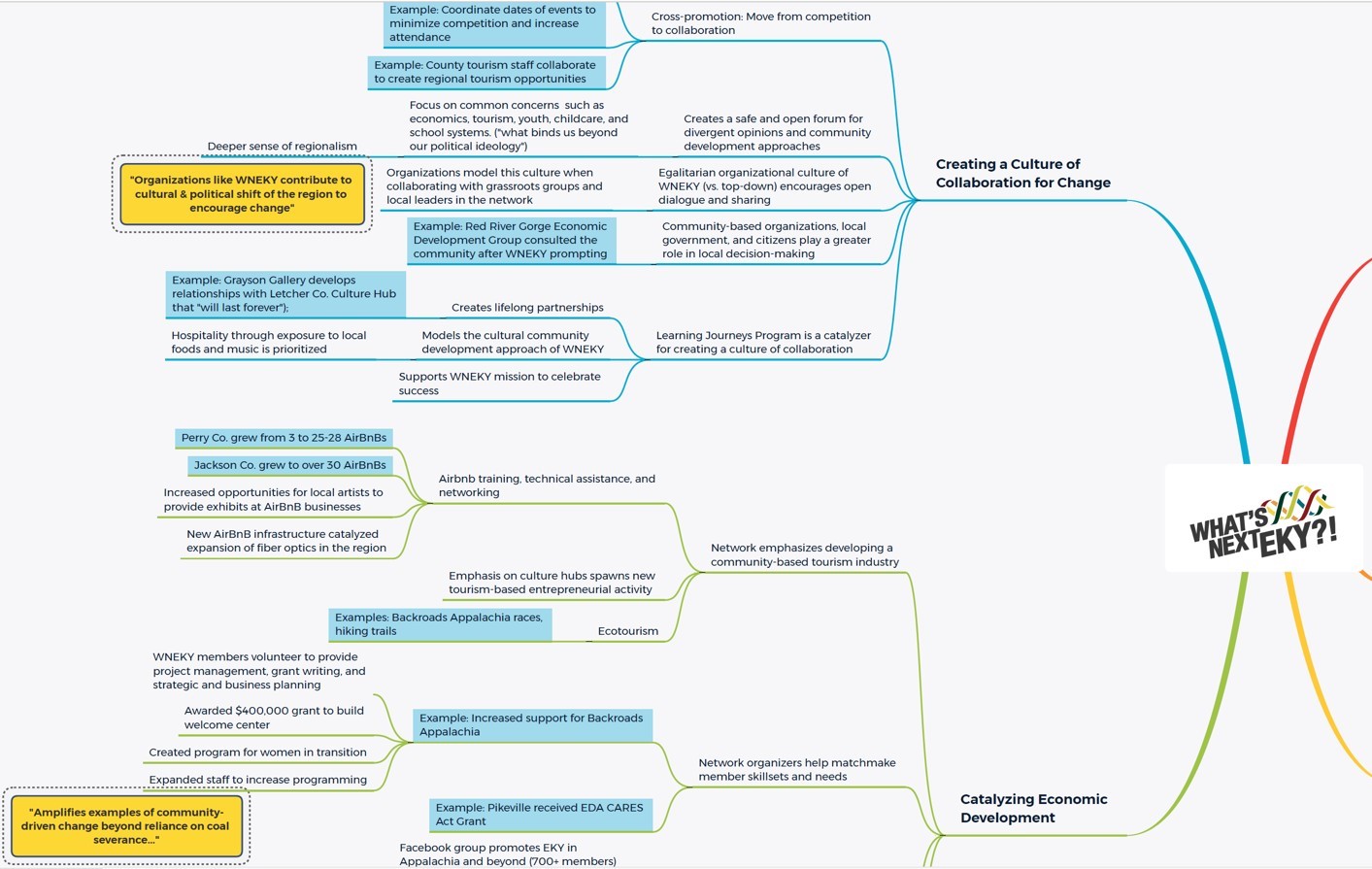The image is a detailed poster chart on a white background, primarily using black text with selective yellow and blue highlights. The chart is designed similarly to a flowchart or table, starting with multiple intertwined categories that converge into one, then branch out again. The main focus is on creating a culture of collaboration for change and catalyzing economic development, with subtopics on cultural and political shifts and examples of community-driven change. The text is small and intricate, organized through numerous brackets, making it challenging to read. The top section emphasizes a blue color scheme, while the bottom is highlighted in lime green, illustrating the different focal points related to economic and cultural transitions, particularly in renewable energy and diminishing reliance on coal severance.